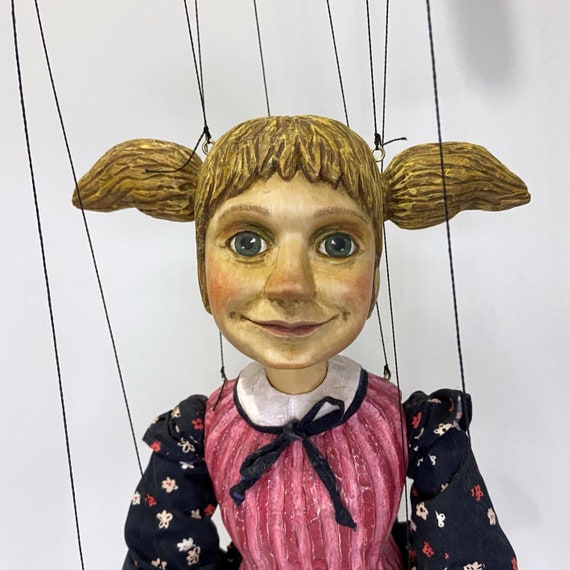In this image, we see a string puppet of a girl with short pigtails that resemble Pippi Longstocking, each sticking out to the sides of her face. Her hair is a dirty blonde shade, and she has shaggy bangs framing her forehead. The puppet features gray eyes, though they appear to have a touch of blue, and she is smiling with her mouth closed. Her cheeks and the tip of her nose are rosy, and there seems to be a hint of reddish eyeshadow on her eyelids.

The girl is dressed in a distinctive outfit: the main body of her dress features vertical stripes in varying shades of pink and fuchsia. The collar area of the dress is white with a dark blue hem, complementing the dark blue bow tied at the front of her chest. Her long sleeves are also dark blue, adorned with an array of flowers in different colors, including peach, white, and red.

Attached to her are numerous strings that control her movements: at least two strings are connected to each pigtail, two at the back of her head, and two for each hand. The intricate detailing and vibrant colors of her dress, combined with the functional strings, bring this wooden puppet to life.